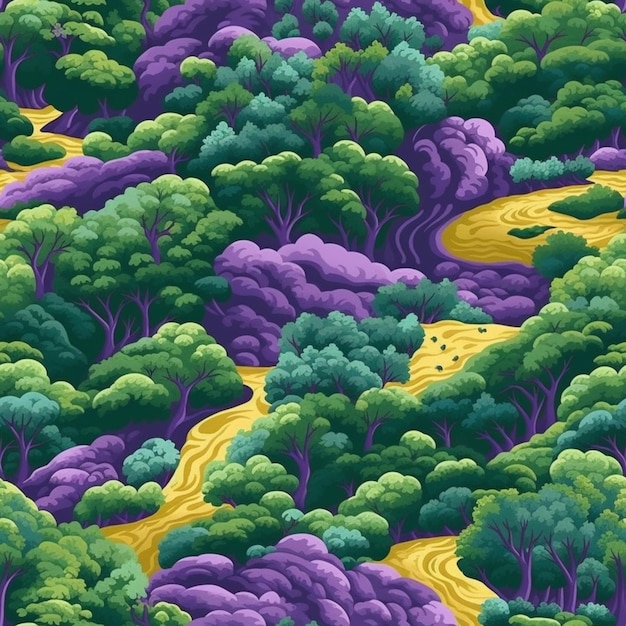This whimsical CGI or cartoon-style illustration depicts a vibrant, surreal forest that is rich in color and detail. The forest is densely populated with predominantly green trees, featuring varied shades of green, from dark to blue-green, and intermixed with trees that have purple trunks or leaves. The trunks of the trees are long and winding, and the entire scene is uniformly illustrated with rounded edges that give it a cohesive, modern look. Purple rocks are scattered throughout the forest floor, adding to the surreal atmosphere.

Flowing through this lush landscape are at least two yellow rivers, each starting in the upper corners of the image – one on the left and one on the right – and meandering downstream. The rivers are depicted with a mixture of dark and light yellow hues, creating a swirling effect that suggests movement. Dark yellow swirls on a lighter yellow background highlight the direction of the water's flow. In the rivers, dark-colored shapes suggest the presence of aquatic creatures, enhancing the dynamic and lively feel of the image. The combination of vibrant colors, elongated tree trunks, and flowing streams evokes a sense of an enchanted, almost Amazon-like rainforest.